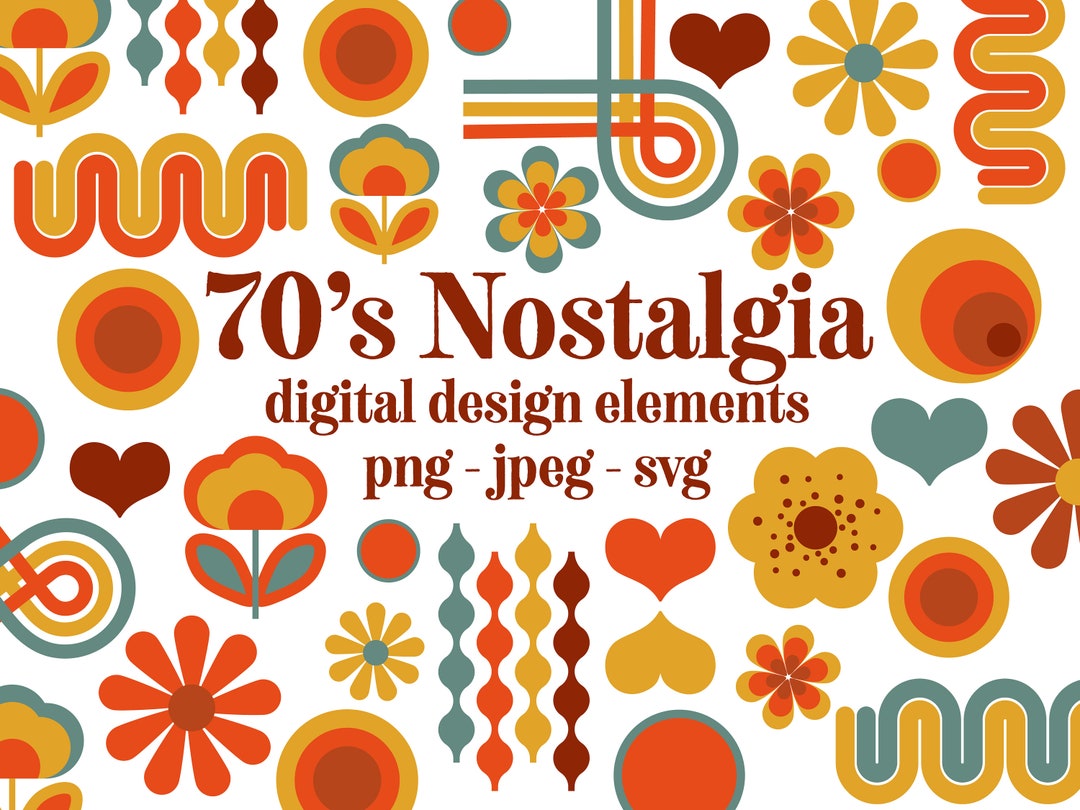The image is of a vibrant poster, predominantly featuring 70s-inspired digital design elements with minimal white space. Centralized in fun, maroon-red text, it reads: "70s Nostalgia Digital Design Elements, PNG, JPEG, SVG." Surrounding this title, the image bursts with iconic 70s art. Predominant hues include teals, yellows, maroons, oranges, gold, and dark red. The artwork includes patterns and symbols characteristic of the 70s era: hearts, whimsical flowers, daisy structures, wavy and curvy lines, intersecting lines, and circles. Notable specific designs include a yellow circle with concentric orange and brown circles, an orange flower with a red center on the bottom left, and another flower profile with green leaves and an orange outline, adorned with orange and yellow petals. This array of vintage motifs encapsulates the nostalgic essence of the 70s.